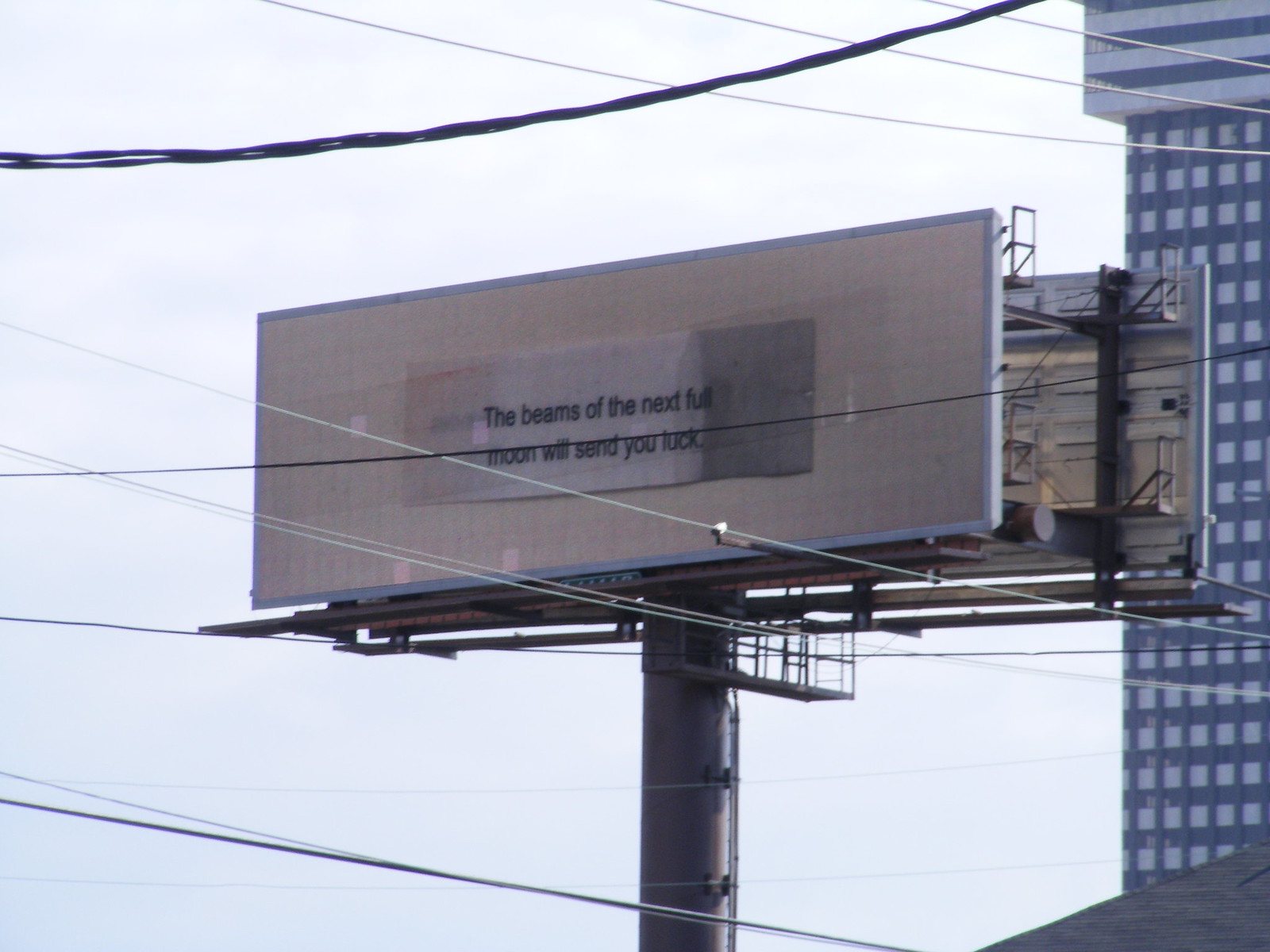This photograph depicts a large billboard prominently positioned against an urban backdrop. The billboard, elevated on a sturdy, cylindrical metal post, features a tan background framed by a gray border. Dominating the center of the advertisement is an image resembling a fortune cookie slip, bearing the message in sans serif font: "The beams of the next full moon will send you luck." This text appears with a bleeding ink effect, adding a touch of sophistication to the otherwise simplistic design.

Surrounding the billboard, a crisscross of electrical cables fills the foreground, contributing to the urban ambiance. A high-rise building with a pattern of black and white stripes is partially visible behind the billboard, juxtaposed against the overcast, light gray sky, indicating a cloudy day. The scene is framed by the geometric harmony of both man-made structures and the chaotic tangle of wires, highlighting the billboard as a focal point in the bustling cityscape.